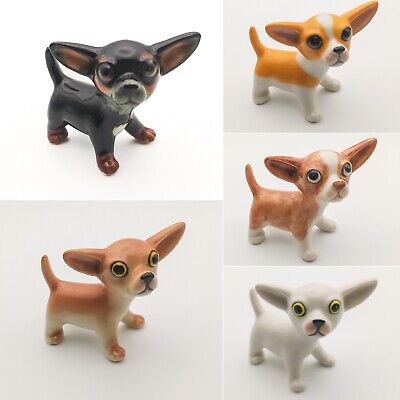This image presents a collection of five photographs depicting small ceramic figures of chihuahuas, all set against a white background. At the top left, a predominantly black figurine with a grey muzzle and large, bulging dark eyes gazes directly at us with its ears extending outward and its tail lifted. Below this is a tan chihuahua figure, similarly styled with long ears and a lifted tail. The top right photograph showcases an orange and white chihuahua, while the middle right features another tan and white chihuahua with dark eyes, looking slightly upwards with a reddish nose. The bottom right displays a plain white chihuahua figure. All these ceramic chihuahuas are characterized by their prominently large, expressive eyes, lifted tails, and detailed features that capture the essence of these adorable small dogs.